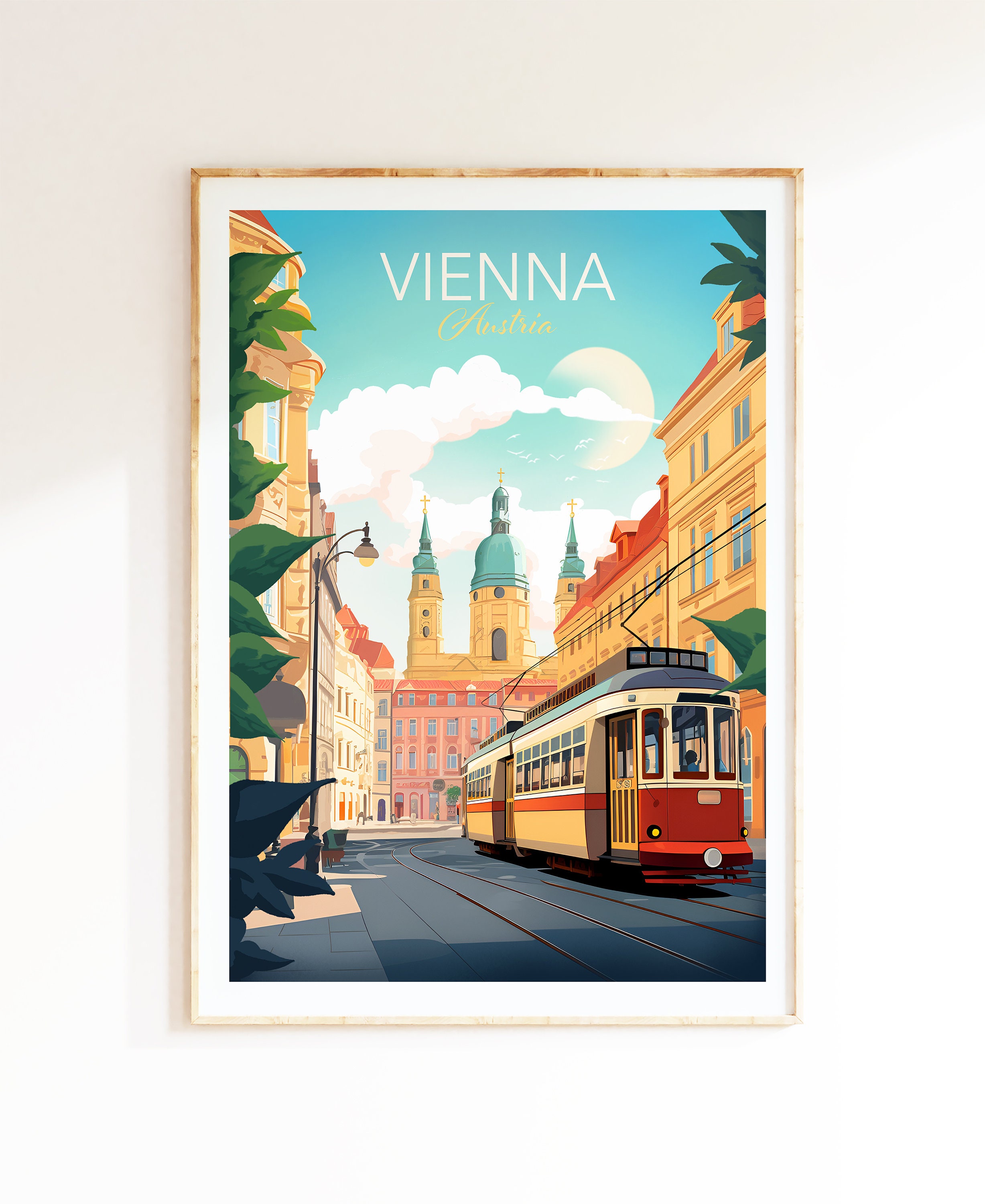This is a detailed travel poster of Vienna, Austria, designed in an Art Deco style and framed in a clipart aesthetic. The sky in the background is a serene blue with puffy white clouds and a celestial body that resembles a moon but suggests daylight. Dominating the center of the sky, the word "Vienna" is prominently displayed in white lettering, with "Austria" written below it in elegant cursive script. Below this, a cityscape unfolds with a variety of tan buildings, some with distinctive blue and red roofs, others topped with steeples and crosses. Among these structures, a notable palace stands out, characterized by a large central tower flanked by two smaller ones, all sporting blue, bell-like tops with decorative finials. 

The bustling street below is lined with old-style European buildings marked by large windows and golden hues. A red-fronted trolley, with gray top and striking red and yellow sides, constitutes the core focal point of the scene, gliding along tracks and connected to overhead power lines. Green leaves frame the edges of the image, offering a touch of natural beauty to the urban view. Overall, this poster artfully captures the charm and elegance of Vienna, inviting viewers to explore its historic streets and grand architecture under a sunny, picturesque sky.